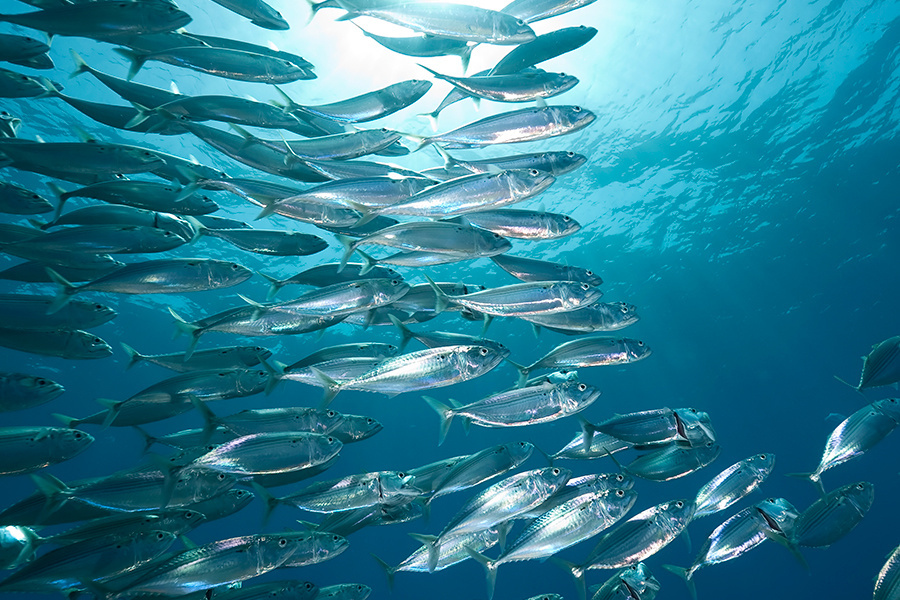This underwater photograph captures a school of silver, shiny mackerel swimming cohesively to the right in the clear, aquamarine water. Taken from beneath the fish, the image displays the sun at the top center, casting a bright light that illuminates the fish, particularly highlighting the ones towards the center and left of the frame while the ones on the right appear darker. The fish, approximately six to eight inches long, are uniformly swimming in the same direction, with their distinct pale stripes visible. The scene includes over fifty fish, if not more, and the upper right quarter of the photograph is devoid of any fish, showing only the clear blue water. The clarity of the water and the focused, synchronized movement of the fish create a mesmerizing and serene underwater tableau.